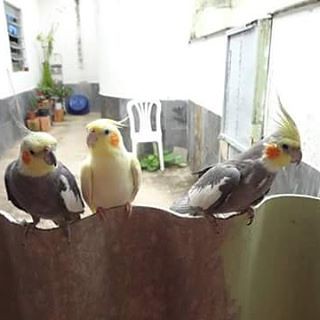The low-quality and small photograph depicts an indoor scene with three budgies perched on a corrugated piece of metal, commonly used for roofing. The setting appears to be a walled patio area or a courtyard. The upper part of the background features a white wall with an open window letting in sunlight. Below the window, the wall has a gray wooden border or fence. On the left side of the background, there are some plants and possibly discarded items like boxes, which are difficult to identify clearly due to the image quality.

In the foreground, the three budgies face the camera. The bird on the right has a predominantly gray body with a notable white patch on its right wing, and an orange spot on the side of its face. Its head feathers are raised upwards at a 45-degree angle. The middle budgie is largely yellow with a prominent orange circle on the side of its face. The left-most bird resembles the one on the right, having a gray body, white wing patch, yellow head, and an orange spot on its face. Their perch consists of a piece of corroded metal that is heavily rusted on the left two-thirds and green on the right side.

In the distant background, besides the white plastic garden chair, one can spot various items including a large basin or bucket along another wall and a sliding wooden door which might lead outside. The entire scene is softly focused, with a blurry and indistinct backdrop, enhancing the prominence of the budgies despite the overall low image quality.